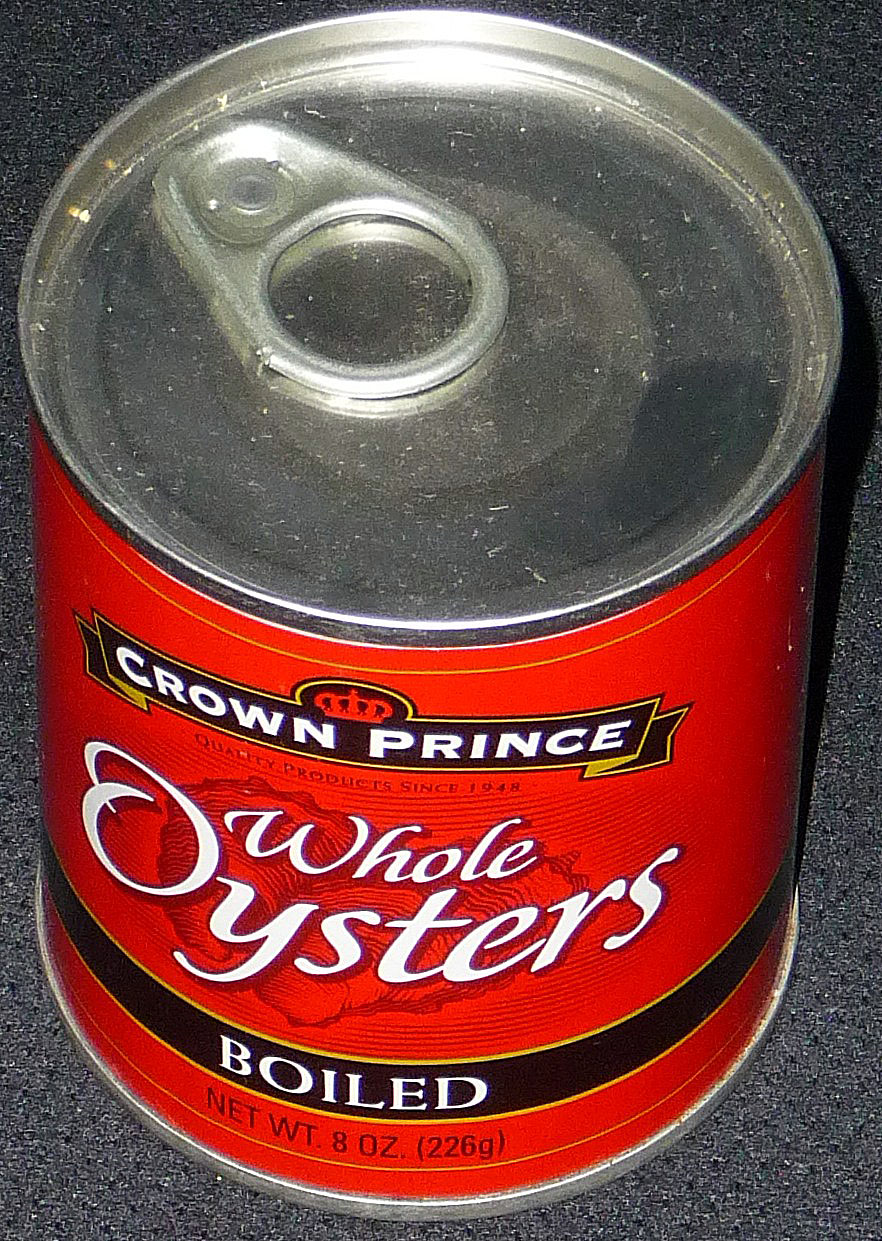The image is a color photograph providing a close-up view of a tin of food that entirely fills the frame. The photograph is taken from a 45-degree angle above the can, allowing the viewer to see the full top surface, including the ring pull tab. The ring pull is flush with the surface, indicating it has not been used, with its rounded part oriented towards the 4 o'clock position and the top part facing the 10 o'clock direction.

The can features a red label with the brand name "Crown Prince" prominently displayed. Beneath the brand name, the label reads "Quality Products since 1948." In stylized, slightly italic white text, it specifies that the contents are "whole oysters," with elegant flicks on the ends of letters such as 'H' and 'W.' Encircling the bottom circumference of the can, there is a black horizontal strip outlined by thinner yellow lines at the top and bottom. Within this black strip, "BOILED" is written in all capitalized white letters. At the very bottom of the label, it states the net weight of the can's contents as 8 ounces (226 grams).